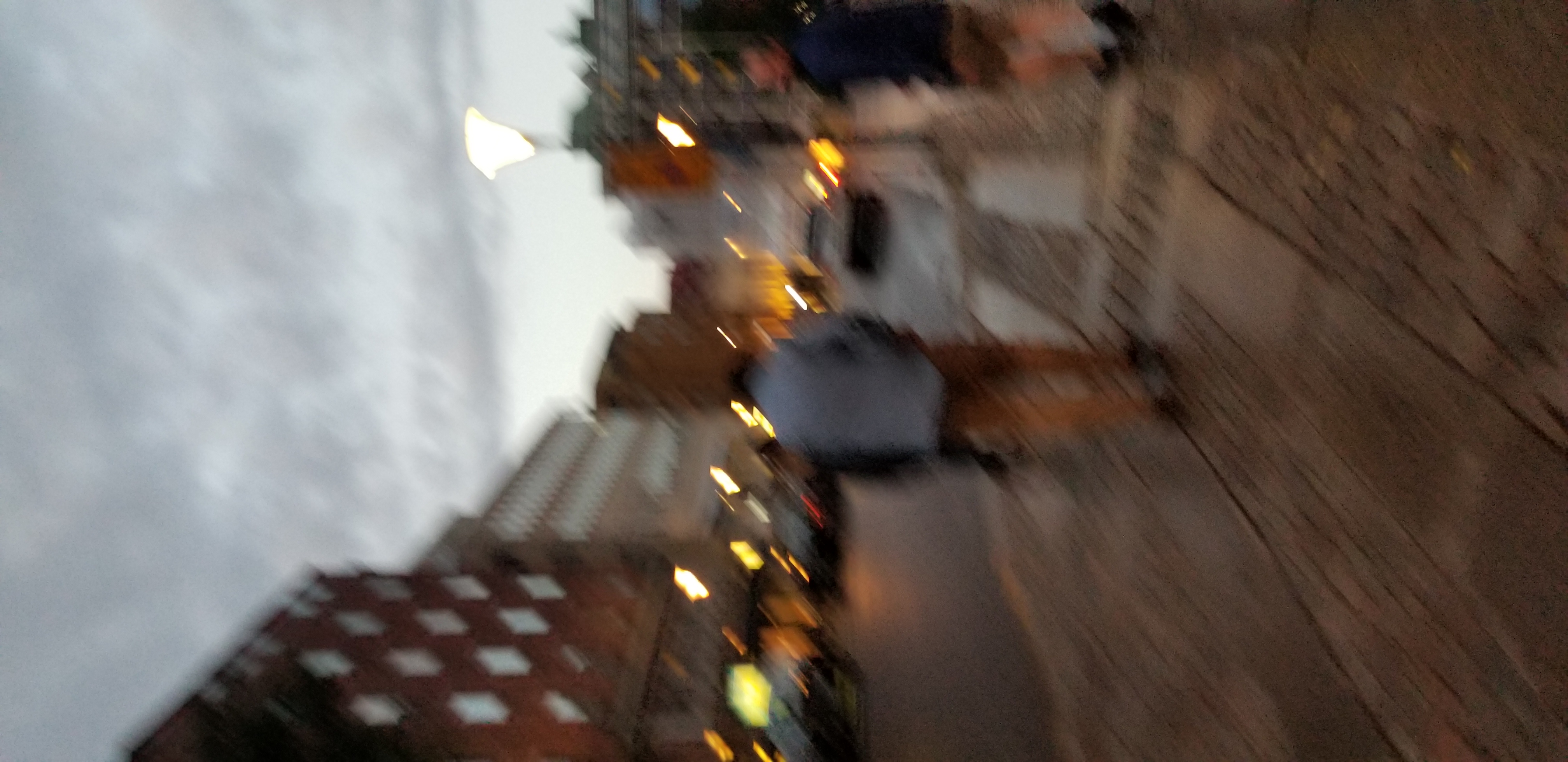This image presents a tilted view of an urban scene, requiring viewers to turn their heads to the left for proper orientation. The foreground features a brown brick walkway, on which two individuals are present. The person on the left is wearing a light blue jacket paired with brown khaki pants, while the person to the right is clad in a dark blue jacket, brown khaki shorts, and black shoes. 

To the left of these individuals, a road is visible with several blurred cars traveling to the left. Adjacent to the road are a series of brown buildings, accompanied by a taller gray building in the background. The upper portion of the image captures a beam of light cutting through an overcast, cloudy gray sky.